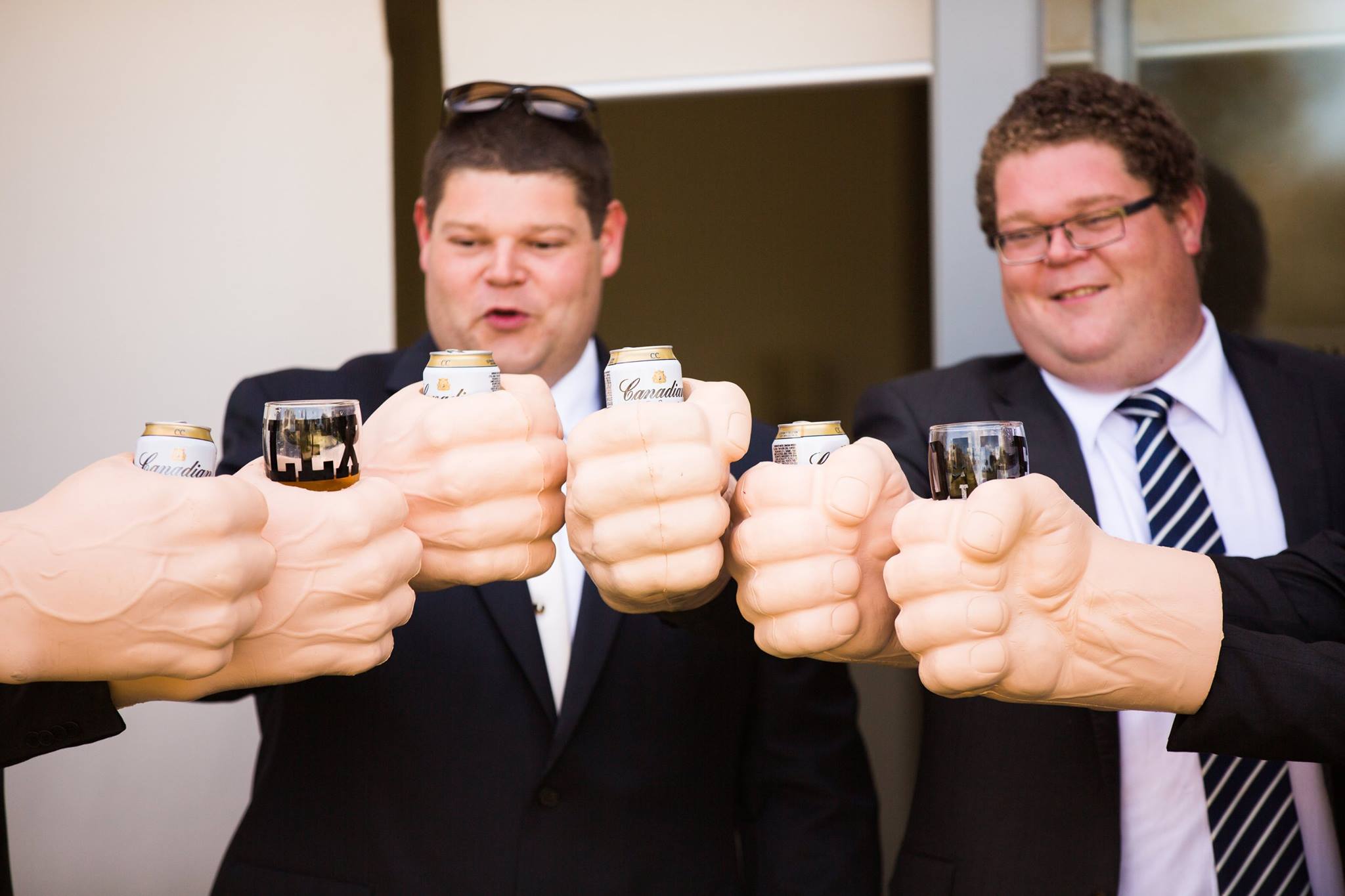In the image, two large men dressed in dark blue suits with white button-down shirts stand prominently in the background. The man on the right, smiling, sports a diagonally striped tie, glasses, short brown hair, and a couple of chins. The man on the left, with sunglasses resting atop his head, also has short brown hair, an open mouth, and multiple chins, though it's unclear if he’s wearing a tie. Centered in the foreground, a semicircle of six artificial, oversized fists grip tiny cans and shot glasses. Each highly detailed fist, complete with visible veins and enlarged fingers, either holds a beverage can—including one partially labeled "Canadian"—or a glass with black writing, one of which reads "Lex" and another "Damn." The setting appears to be indoors, possibly at a party or meeting, underlined by the visual emphasis on the surreal, plastic-like hands forming a striking contrast against the suited men.